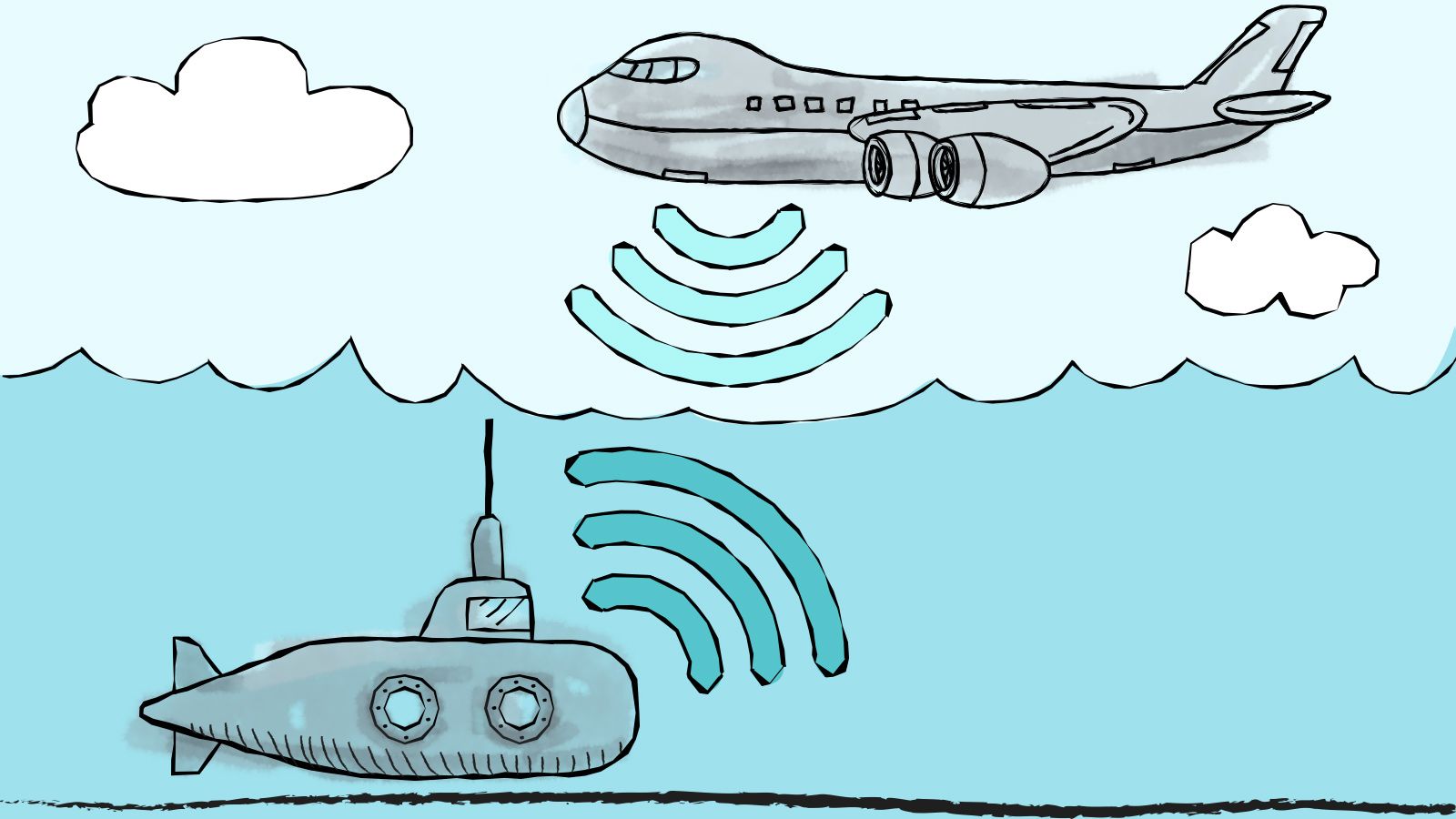A beautifully detailed drawing depicts a serene scene transitioning from the sky to the ocean. The top portion of the image features a light blue sky with two fluffy clouds on the left and one on the right. Above the cloud on the right, a gray airplane is depicted, emitting three downward-pointing lines that symbolize signals. Below this sky scene, the deeper blue ocean hosts a gray submarine, complete with an antenna on top. The submarine emits three diagonal lines ascending toward the airplane's signals, suggesting a communication link between the two vehicles. This illustration eloquently captures the theme of inter-vehicular communication across different mediums.